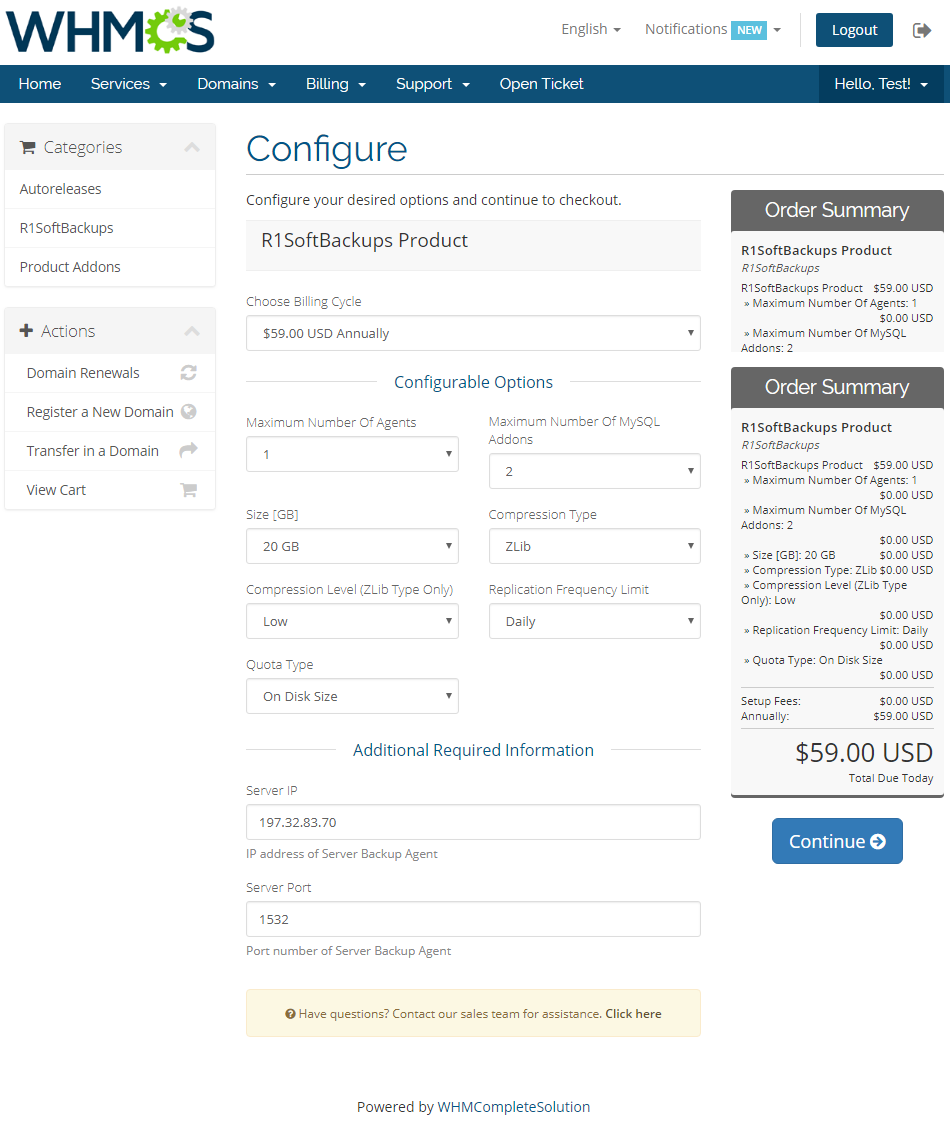This is a detailed screenshot of the WHMCS website's configuration page. Its logo features the letter "C" styled to resemble a green screw, complemented by a smaller gray screw on top. The interface includes a navy blue header at the bottom of the title, organizing navigation links in a row: "Home Services" with a down arrow, "Domains" with a down arrow, "Billing" with a down arrow, "Support" with a down arrow, and "Open Ticket." There is also a logout button and a "Hello Test" button on the same header row.

The current page is the "Configure" section, offering a choice for the billing cycle priced at $59 USD annually. The "Configurable Options" section features seven drop-down menus: "Maximum Number of Agents," "Size," "Compression Level" set to low, "Coda Type" set to "Disc Size," "Maximum Number of MySQL Add-ons" set to 2, "Compression Type" set to "Zlib," and "Replication Frequency Limit" set to daily.

Additionally, the "Additional Required Information" section requests a "Server IP" and "Server Port," which is 1532. At the bottom of the page, a yellow rectangular box offers assistance, reading, "Have questions? Contact your sales team for assistance. Click here."

On the right side, there are two "Order Summary" boxes. The first is brief, whereas the second provides detailed information, culminating in a total cost of $59 USD. Beneath this summary, there is a blue "Continue" button.